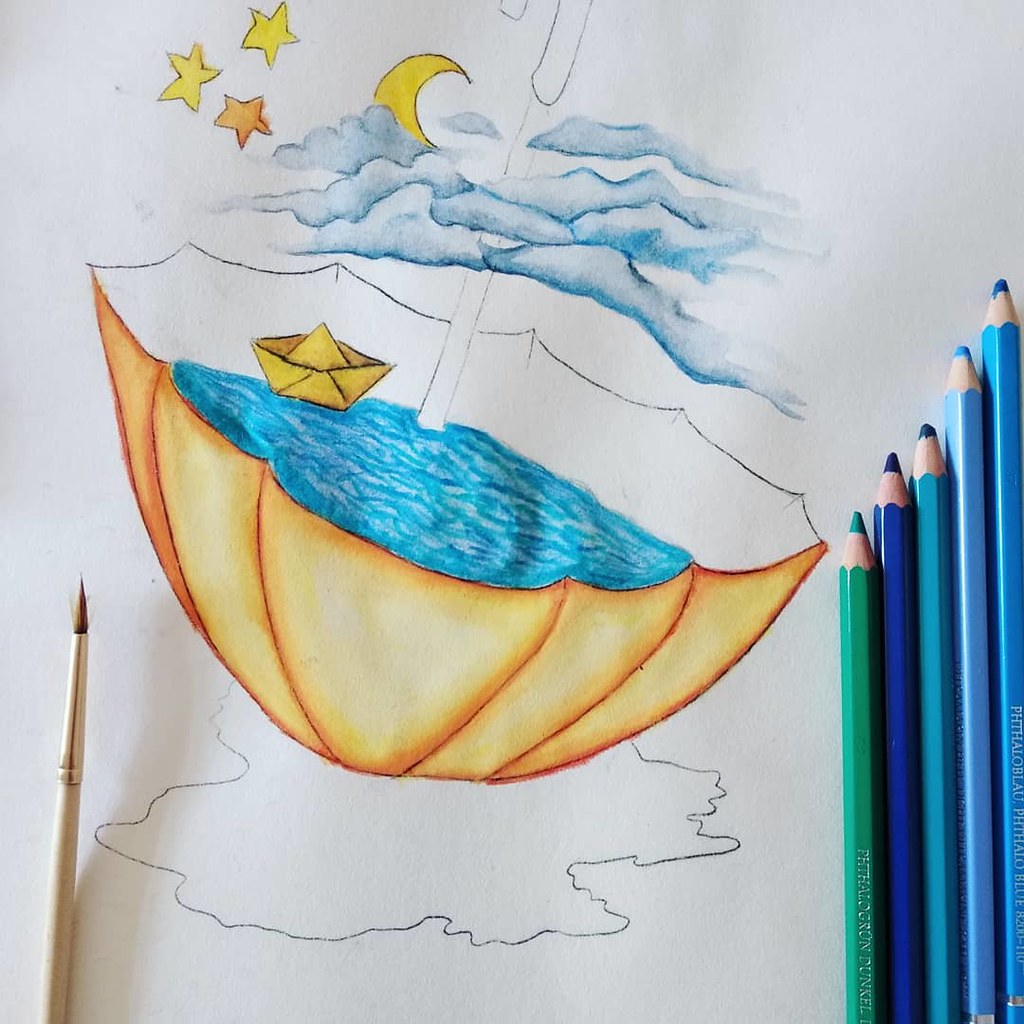This top-down view showcases a meticulously completed piece of artwork created using watercolor pencils. The central theme is an inverted umbrella filled with water, sheltering a small paper boat. The backdrop is a nocturnal sky adorned with blue clouds, hastily drawn stars, and a crescent moon partially obscured by clouds. The umbrella's exterior is an orangey-yellow hue, while the paper boat mirrors a vibrant yellow shade. Situated at the bottom left of the image is a paintbrush, and on the right, a set of five watercolor pencils in varying heights, ranging in color from teal-green to light blue, are neatly arranged.